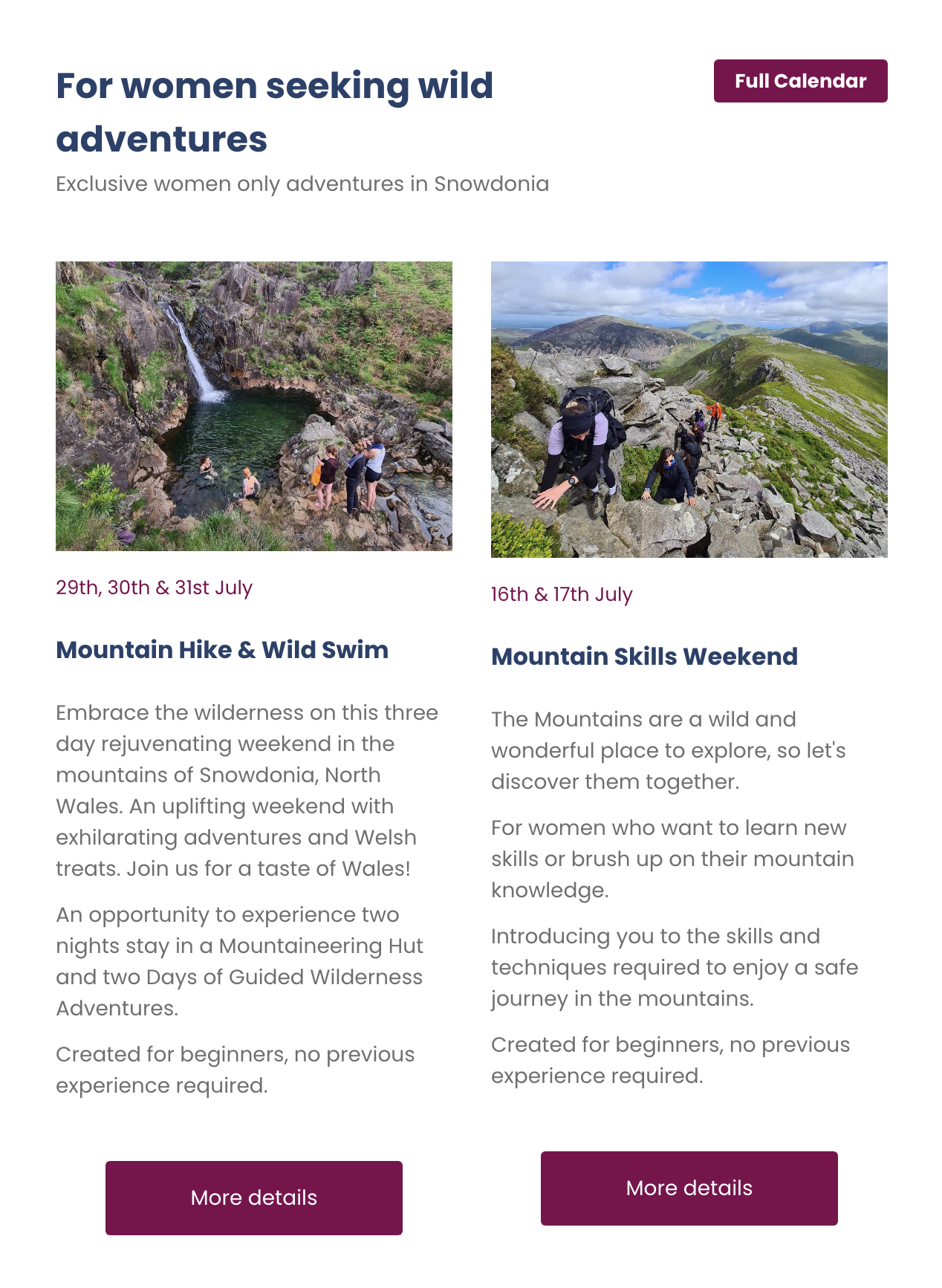The webpage, designed with a minimalist white background, features a prominent blue heading that reads "For Women Seeking Wild Adventures." In the top right corner, a maroon box labeled "Full Calendar" offers navigational aid. Under the main heading, it advertises "Exclusive Women Only Adventures in Snowdonia."

Accompanying the text are two engaging images, each with corresponding descriptive columns. The first image on the left showcases a scenic grotto with a waterfall surrounded by people. Below this image, the caption highlights a 3-day event scheduled for July 29th-31st, featuring a mountain hike and wild swim in the mountains of Snowdonia, North Wales. It invites participants to "embrace the wilderness" and promises an "uplifting weekend" with exhilarating adventures and Welsh treats. It emphasizes an immersive experience with two nights of accommodation and two days of guided wilderness adventures, tailored for beginners with no previous experience required. A maroon box at the bottom offers additional details.

The second column to the right corresponds with an image of people engaged in a mountain hike. It describes an event on the 16th and 17th of July, focusing on "mountain skills." The text calls the mountains "a wild and wonderful place to explore" and encourages women to discover them together. It is aimed at teaching new skills or refreshing existing mountain knowledge, ensuring a safe journey. As with the previous event, this is also designed for beginners with no prior experience needed.